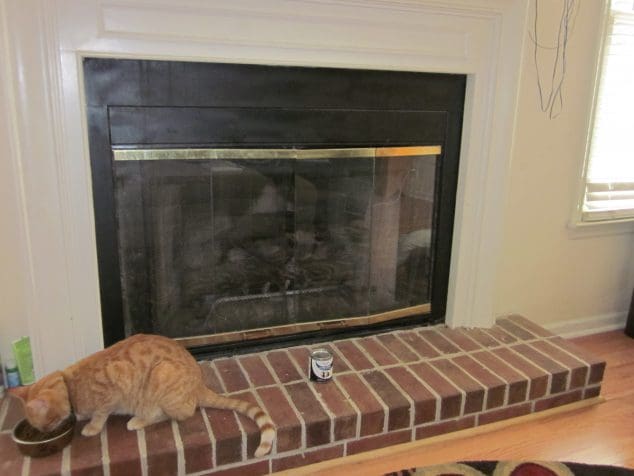The photograph captures an indoor scene featuring a prominently white-painted fireplace mantel set into a similarly white wall. The fireplace itself has a glass front, revealing a black and gold inset typically associated with gas fireplaces. Positioned in front of the fireplace is a small red brick step up from a light brown wooden floor. To the right, a white-framed window with open white blinds allows sunlight to pour in, illuminating the room. An orange cat with dark orange stripes is focused on eating from a silver bowl placed on the brick surface. Directly behind the cat, a can of cat food lies on the brick step. The room's baseboards are white, providing a clean contrast to the neutral tones of the wooden floor and the subtle tan undertone described in the wall color. On the bottom right edge of the image, there is a faint glimpse of what might be a piece of furniture or a rug.